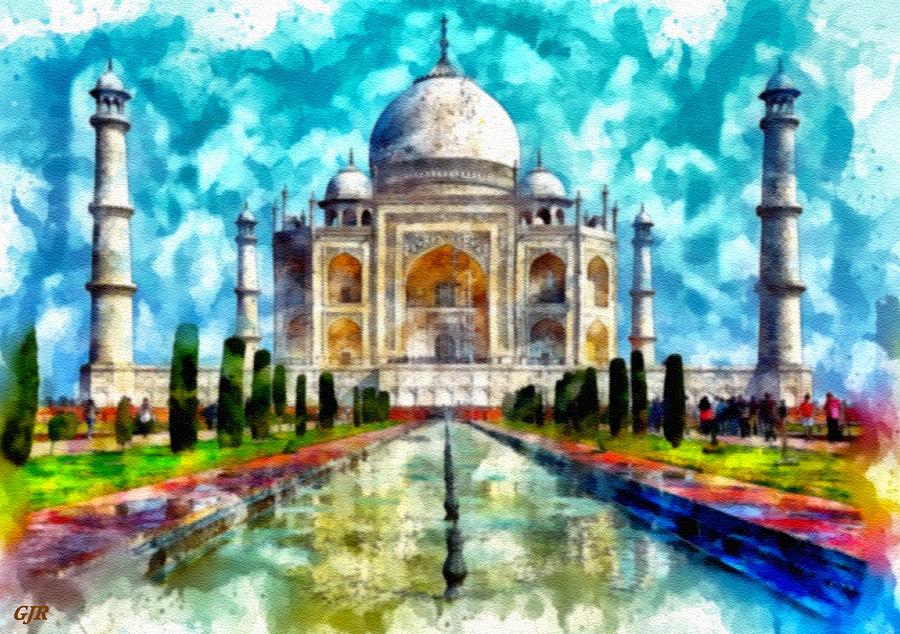This detailed watercolor or digital painting vividly captures the iconic Taj Mahal in India. The sky is a striking and vivid blue, creating a beautiful backdrop for the symmetrical scene. The majestic white structure of the Taj Mahal, with its large central dome flanked by two smaller domes, stands prominently. Two tall, slender towers rise on each side of the building, resembling watchtowers or lighthouses. 

A long reflecting pool stretches down the center of the image, with the calm water reflecting the grandeur of the Taj Mahal. The pool's water shimmers with shades of green, yellow, and gold, adding depth and color. Flanking the pool, there are red walkways and lush, green lawns dotted with tall, thin bushes and trees, creating a symmetrical balance. The scene is adorned with various hues, including reds, yellows, and blues, enhancing the vibrancy of the painting. Sidewalks lead toward the magnificent structure, where you can even spot tiny figures of people walking around, adding a sense of scale and life to the tranquil setting.